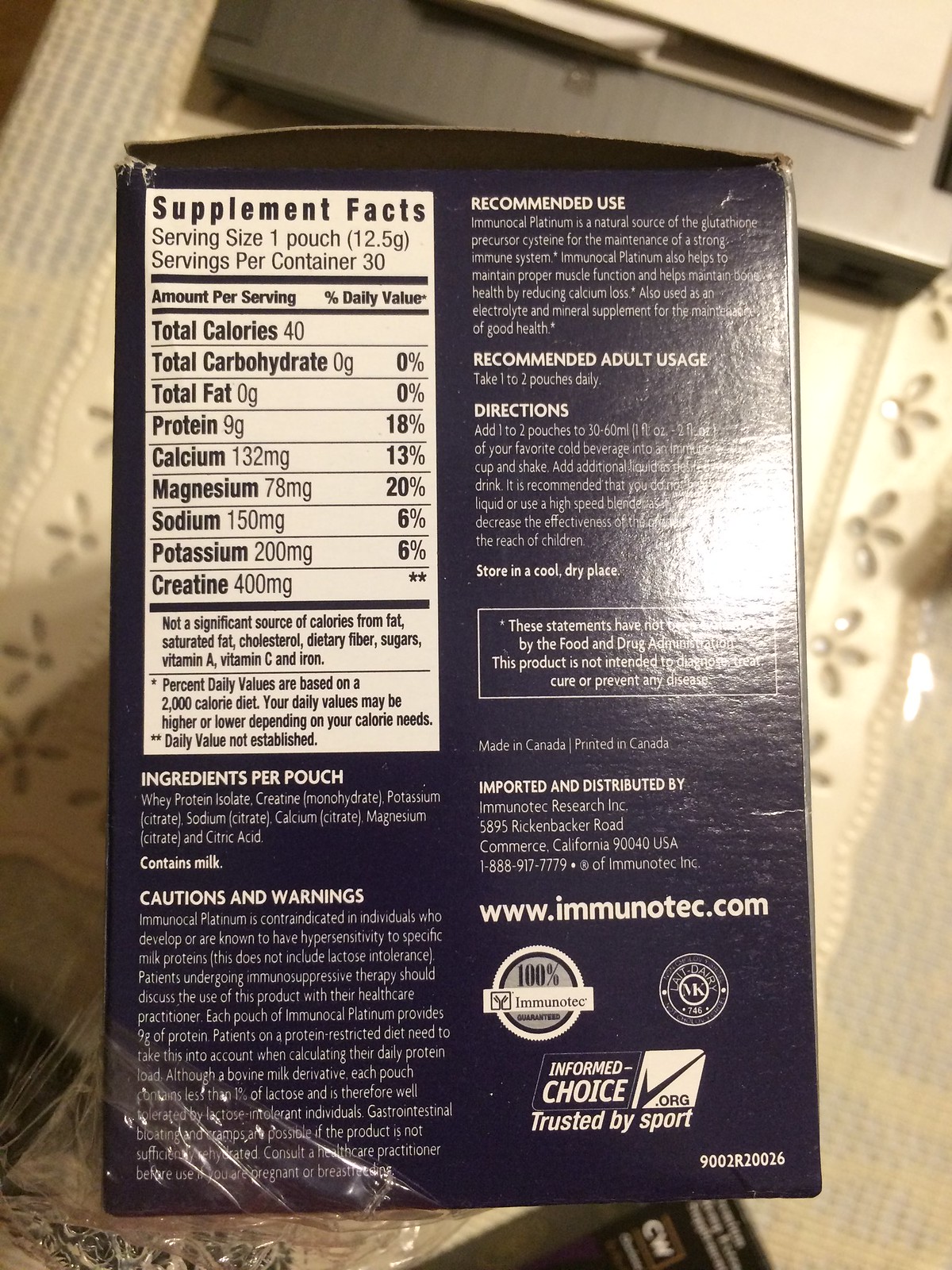The image depicts the nutritional information and packaging details of a product called "Immunitech". The package is dark blue with white lettering. At the top right corner, there is a detailed section titled "Supplement Facts". It specifies that a serving size is one pouch weighing 12.5 grams, with 30 servings per container. 

Nutritional values per serving include:
- Total calories: 40
- Total carbohydrates: 0g, 0% Daily Value
- Total fat: 0g, 0% Daily Value
- Protein: 9g, 18% Daily Value
- Calcium: 132mg, 13% Daily Value
- Magnesium: 78mg, 20% Daily Value
- Sodium: 150mg, 6% Daily Value
- Potassium: 200mg, 6% Daily Value
- Creatine: 400mg

A disclaimer notes that the product is not a significant source of calories from fat, saturated fat, cholesterol, dietary fiber, sugars, vitamin A, vitamin C, and iron. The values provided are based on a 2000-calorie diet.

Below this, the ingredients per pouch are listed as whey protein isolate, creatine monohydrate, potassium citrate, sodium citrate, calcium citrate, magnesium citrate, citric acid, and contains milk. There is also a caution and warning section with a long disclaimer.

On the left-hand side of the package, the "Recommended Use" section is outlined, though the small print is hard to read due to glare. This section includes:
- Recommended adult dosage: Take one to two pouches daily.
- Directions: The specific instructions are obscured by glare.
- Store in a cool, dry place.

Further information is provided in a box stating that the product is made and printed in Canada. It is imported and distributed by Immunotech Research, Inc., located at 5895 Rickenbacker Road, Commerce, California 90040, USA. The contact phone number is 1-888-917-7797. Additionally, the package features the registered symbol of Immunotech, Inc., their website www.immunitech.com, and various logos including the Immunotech logo.